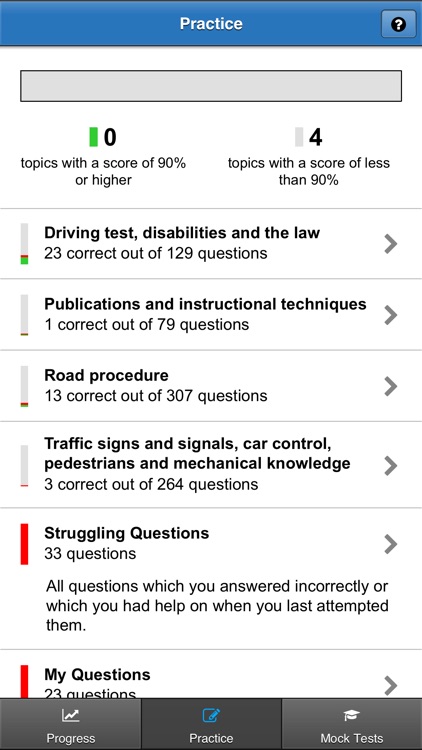This vertical mobile screenshot features a blue header bar at the top, displaying the word "Practice" in the center and a question mark icon on the right-hand side. Below the header is an empty gray horizontal box. Following this, a section outlines performance statistics: "0 topics with a score of 90% or higher" and "4 topics with a score of less than 90%".

The screenshot is from either a car-related app or settings menu. It lists multiple headings in bold font that progress downward, including:

- **Driving Test**
- **Disabilities and the Law**
- **Publications and Instructional Techniques**
- **Road Procedure**
- **Traffic Signs and Signals**
- **Car Control**
- **Pedestrians and Mechanical Knowledge**
- **Struggling Questions** (marked with a red vertical bar on the left)
- **My Questions** (also marked with a red vertical bar on the left)

Each section is accompanied by a gray arrow pointing to the right.

At the bottom of the image, there is a dark gray and light gray bar divided into three buttons:

- The left button reads "Progress."
- The center button reads "Practice," highlighted with a blue pilot icon.
- The right button reads "Mock Tests."